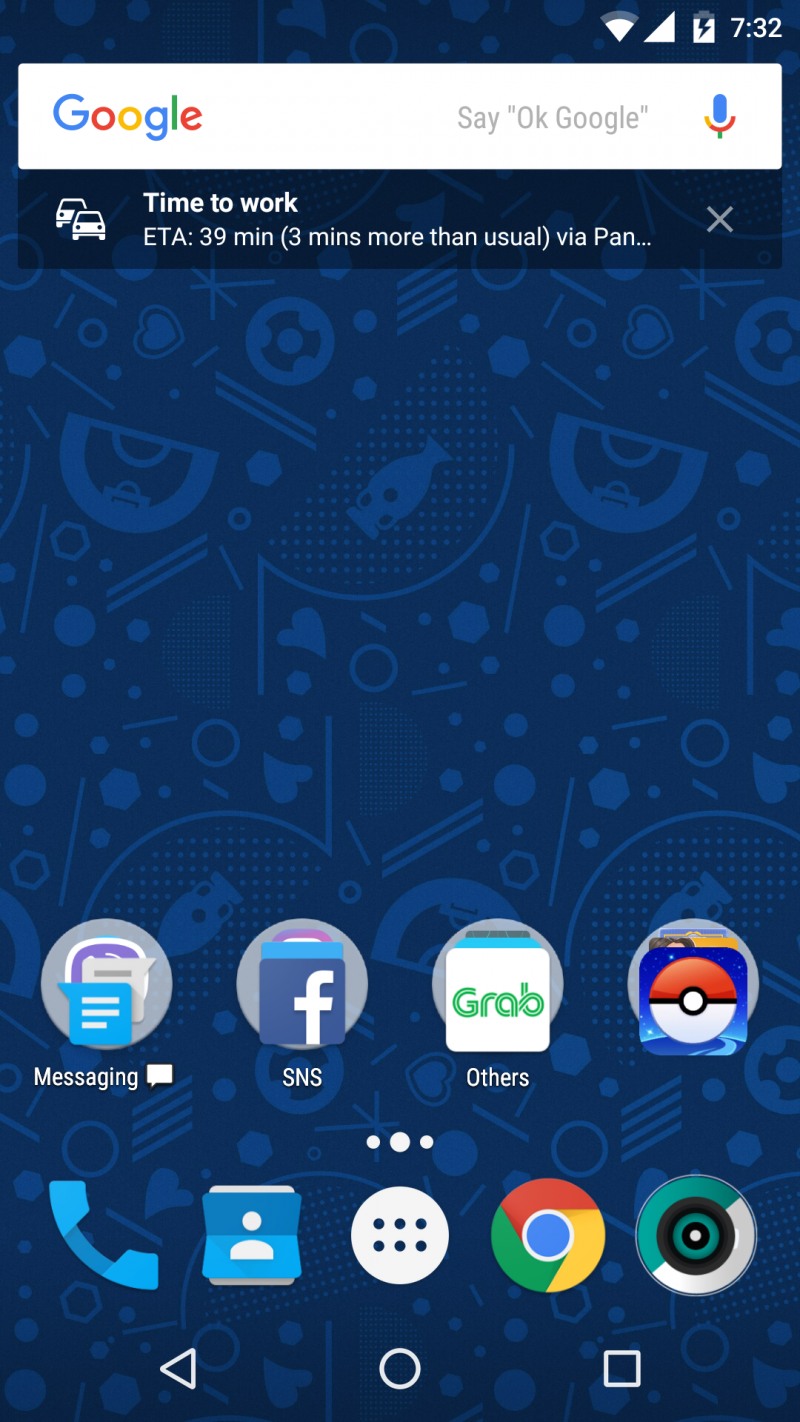Screenshot of a cell phone home screen featuring a complex and visually busy dark blue wallpaper adorned with light blue icons including circles, hexagons, bottles, gears, bags, hearts, and other simple graphics. The top status bar displays a Wi-Fi icon with three out of four signal bars, full cellular signal strength, and an 85% battery charge. The time is shown as 7:32.

Directly below the status bar is a Google search bar, showcasing the Google logo to the left, the phrase "OK Google" in quotes to the right, and a microphone icon. Beneath the search bar, there's an alert featuring an estimate for time to work: "39 minutes" with two cars symbol, and a note indicating it's "3 minutes more than usual via PAN..." with an 'X' option to close the alert.

At the bottom of the screen are four preferred apps alongside a standard dock of five additional apps. The preferred apps include Messaging, SNS, Facebook, and Grab—all clustered together. Additional notable apps in clusters include Pokemon Go. The standard bottom dock comprises a phone icon, a contacts (Rolodex) icon, a 3x2 grid of dots, Google Chrome, and possibly a camera icon.